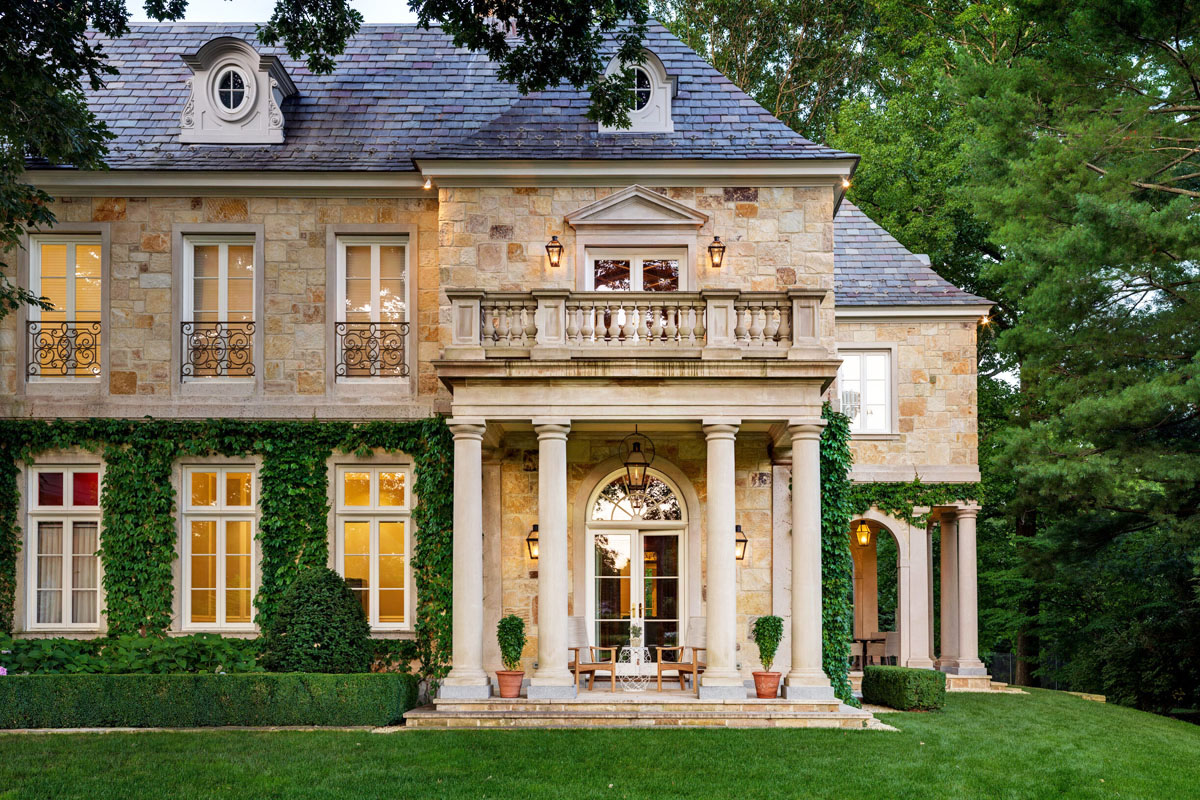The image depicts a substantial, old-fashioned yet well-maintained, brick house that could be considered a mansion. The house appears to be at least two stories tall, potentially three, as it features a small balcony and two small circular windows at the top, possibly part of an attic. The bricks are a combination of yellow, brown, and orange hues, giving the house a warm, inviting appearance. The roof is adorned with blue tiles and includes gables with oval windows.

The front or back entrance is marked by a set of two small steps leading up to a doorway flanked by columns. There are houseplants and potted plants near the entrance, adding a touch of greenery. Several tall windows without shutters adorn the facade, allowing ample daylight to stream in, suggesting a bright, sunny day. The lower level is covered with vines, contributing to the house’s old-fashioned charm.

Surrounding the house is a lush, well-kept lawn with patches of grass and sporadic weeds clinging to the side of the building. To the left side, there is a bush and a hedge, and numerous trees frame the scene, providing a verdant background. There are also small benches in front of the house, further enhancing its picturesque and inviting appearance.